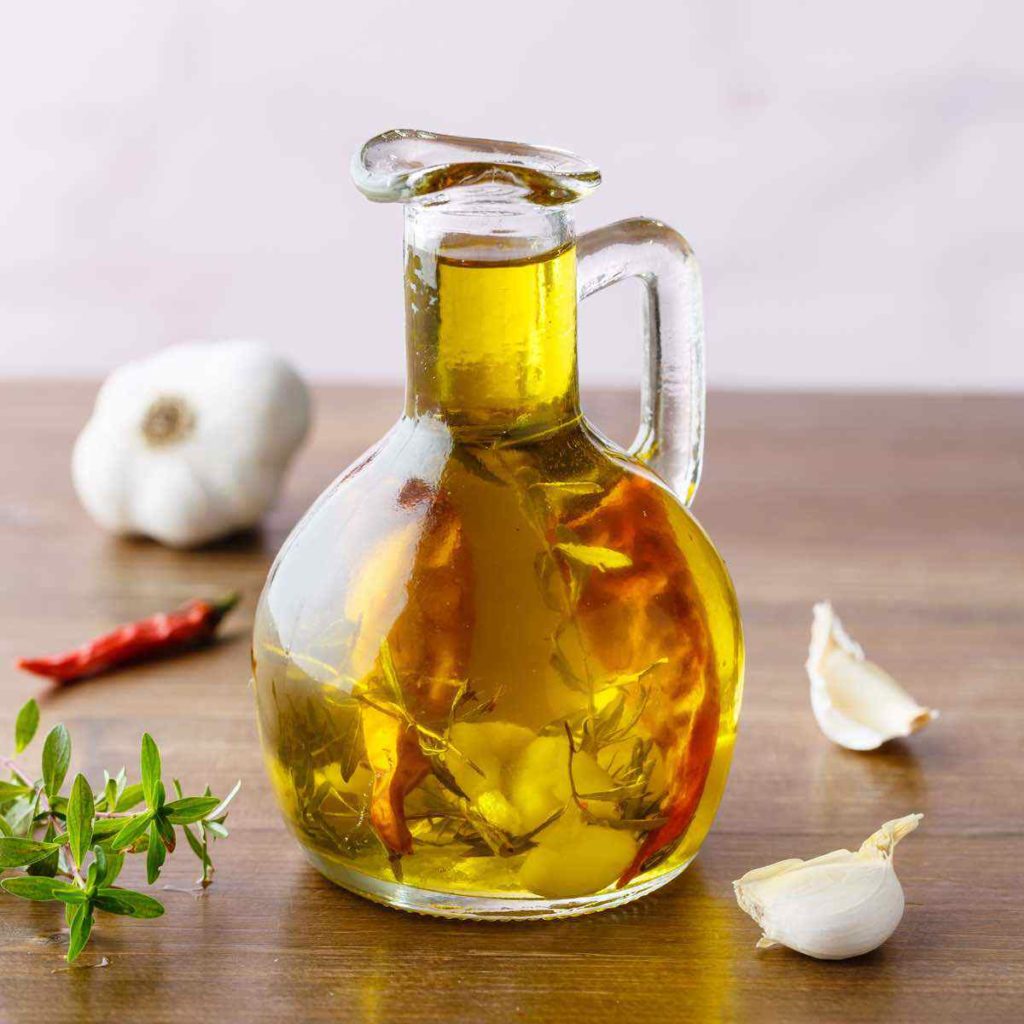This photograph captures a small glass jug, likely filled with olive oil, positioned at the center of a wooden table with a white wall serving as the backdrop. The oil, tinged a dark greenish-yellow, is infused with several aromatic ingredients: garlic cloves, sprigs of rosemary, thyme, two red ancho chilies, and whole black peppercorns. These elements are all visible within the jug. Surrounding the jug on the table are two garlic cloves to its right, while a whole garlic bulb sits in the slightly blurred background, next to a sprig of rosemary and another ancho chili. The focus of the image is clearly on the jug and its rich, infused contents, showcasing the key flavors: rosemary, garlic, and chili.